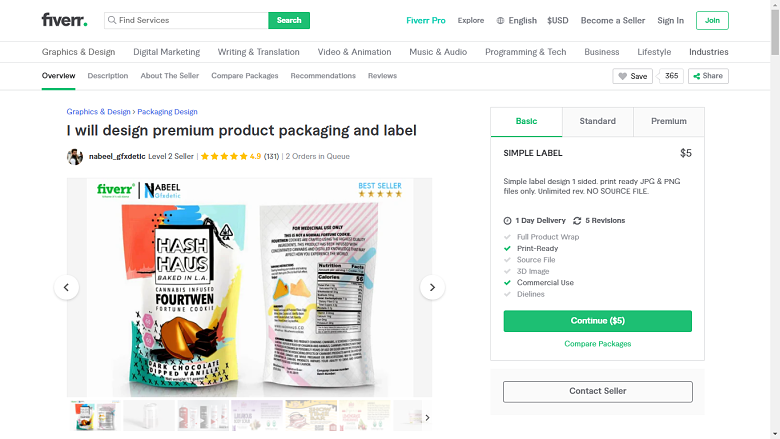**Detailed Image Caption:**

The image depicts the homepage of "Fever," which features a sleek and clean interface with a white background. In the upper left corner, the word "Fever" is displayed in black text, immediately followed by a prominent search bar labeled "Find Services." To the right of the search bar is a green rectangular button with white text that reads "Search." 

To the center right of the page, "Fever Pro" is highlighted in green text. Adjacent to it, in black text, are navigation options for "Explore," "English," and "US dollars," followed by hyperlinks that say "Become a Seller," and "Sign In." There is also a green-outlined rectangle with green text that reads "Join."

Directly beneath this top navigation menu, there is a horizontal list of categories, spanning from left to right: "Graphics and Design," "Digital Marketing," "Writing and Translation," "Video and Animation," "Music and Audio," "Programming and Tech," "Business," "Lifestyle," and "Industries."

Another row beneath features navigational tabs: "Overview" (which is underlined in green to indicate it's the current selection), "Description," "Seller," "Compare Packages," "Recommendations," and "Reviews."

To the right side of the image, there are three rectangular buttons labeled "Save," "$365," and "Share."

The central part of the image shows an eye-catching image of multicolored fortune cookies with a label that reads, "I will design premium product packaging and label." The product depicted is "House Baked in LA Fortwin Fortune Cookies," showcasing both the front and back of the packaging.

To the right of this product image, three rectangular tabs are displayed at the top, labeled "Basic," "Standard," and "Premium." Below these tabs, there is a detailed description in black text outlining the service options: "Simple Label," "Sample Label Design," "One-Sided," "Print-Ready," "JPEG and PNG Files Only," "Unlimited," "No Source File," and "One-Day Delivery."

At the bottom of this section, there is a button labeled "Continue" followed by a visible price tag. Below this button, another option to "Contact" completes the descriptive layout.

This complete and detailed homepage showcases a range of services and categories, providing a user-friendly interface designed to simplify navigation and enhance the user experience.